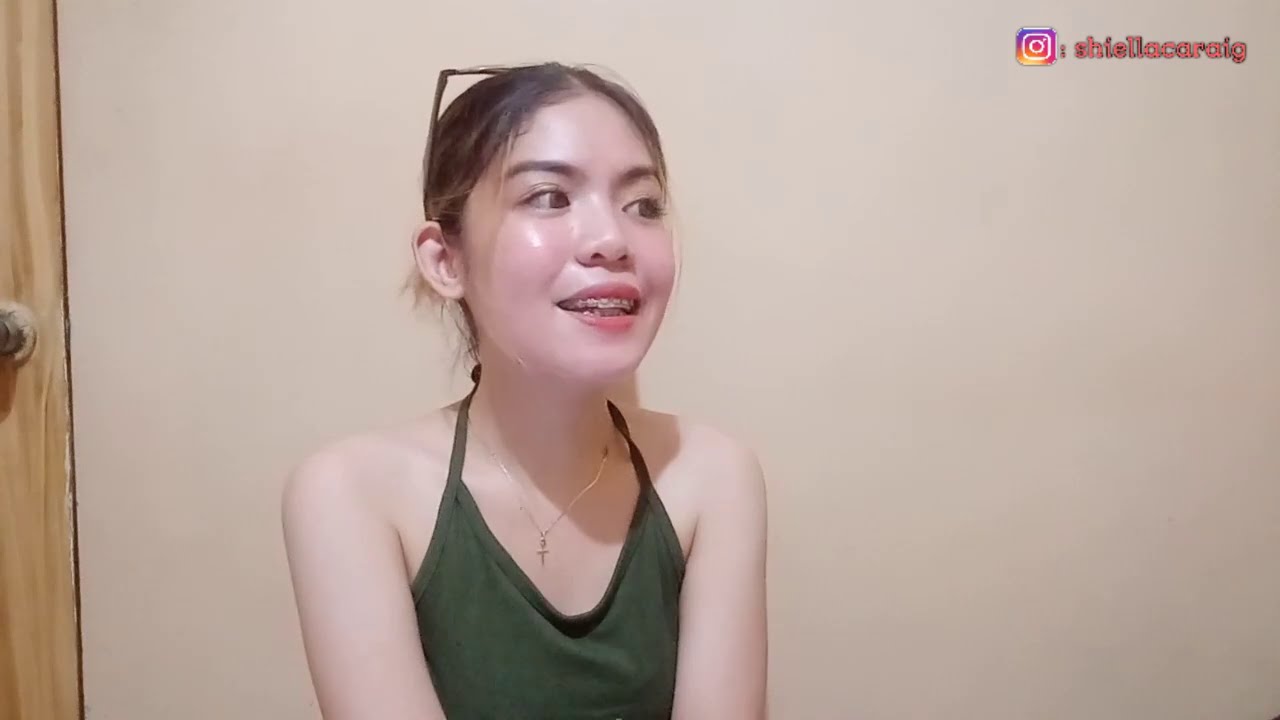The image features a young girl, likely a teenager of Asian descent, seated and facing slightly to the right, with the cut-off point of the photo just below her chest. She has dark, possibly black hair that is parted in the middle and pulled back, adorned with a pair of sunglasses resting on top. Her complexion is very pale, with dark eyes, dark eyebrows, and lips of a pinky coral hue. She appears to be wearing braces and is slightly smiling. Her attire includes a green top that ties behind her neck and is accessorized with a gold cross necklace resting on her chest. The background consists of a light gray or white wall, with part of a wooden door and doorknob partially visible on the left side of the image. In the top right corner, there is an Instagram symbol and some red text, including what appears to be the name "Sheila Caraig."